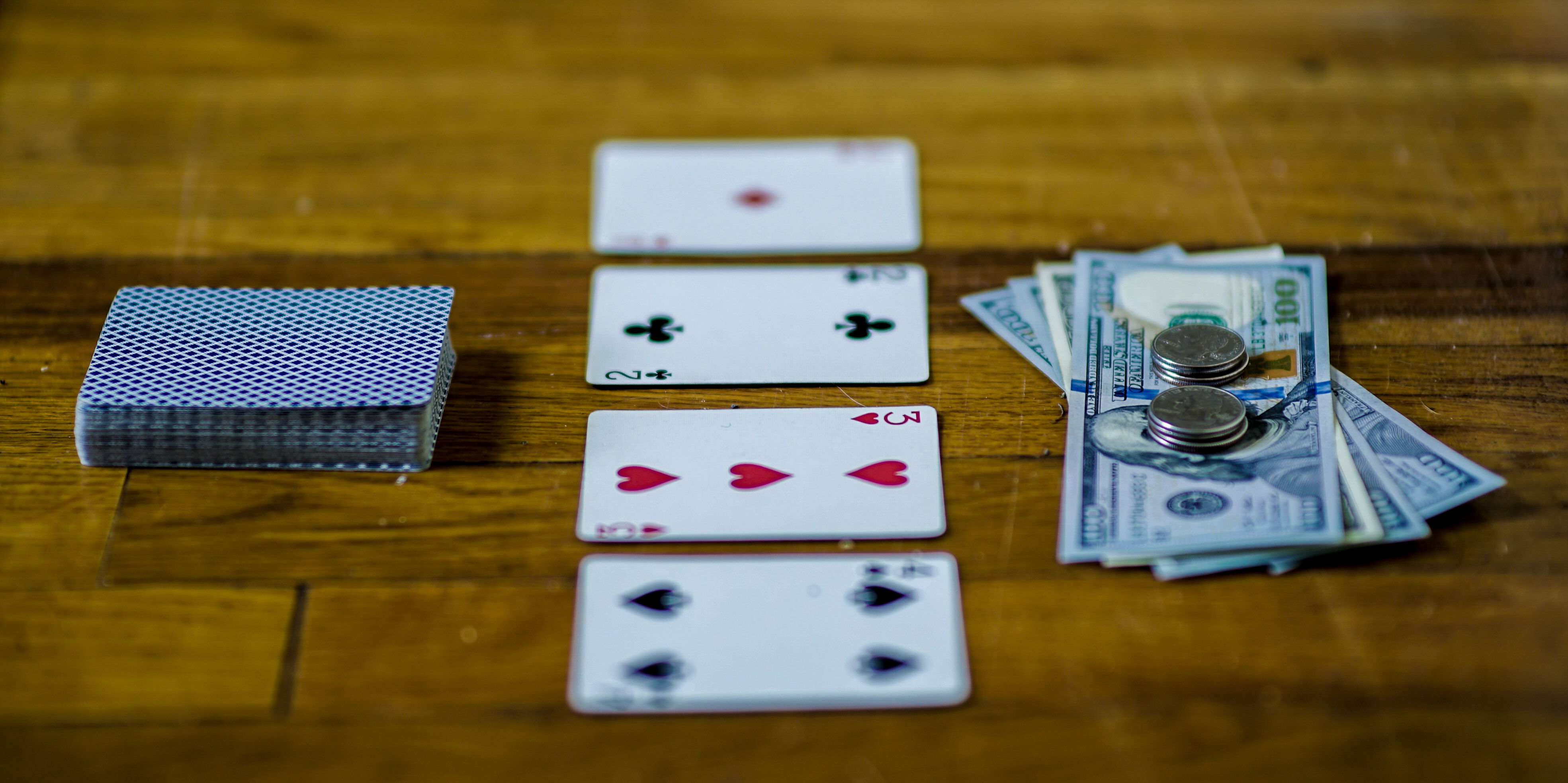A light-medium brown wooden table appears to be the setting for a gambling scene. In the center, a slightly disorganized stack of money is visible, consisting of four or five $100 bills. On top of this stack are two piles of quarters. To the side, there is a blue and white checkered deck of cards with four cards laid out horizontally between the money and the deck. The cards are as follows: a red Ace of Diamonds, a black Two of Spades, a red Three of Hearts, and a black Four of Clubs. The deck of cards is neatly arranged, whereas the stack of money is slightly uneven, with the edges of the bills not perfectly aligned. The image is a bit blurry, adding to the dynamic nature of the scene.